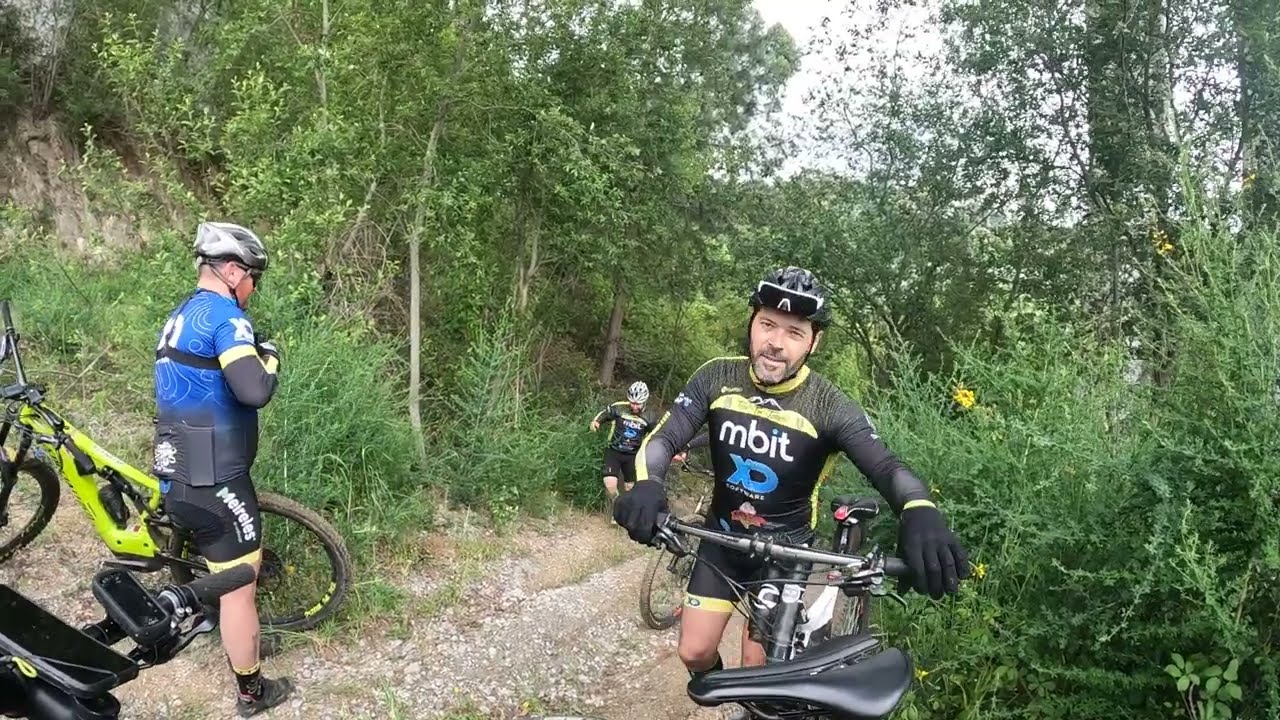In this outdoor scene, three mountain bikers, likely in their late 30s to early 40s, are taking a break on a gravel trail that winds through a rough scrubland area, surrounded by bushes and a few trees with saplings on the right. The trail slopes slightly upward to the left. All three riders are equipped with mountain bikes and are donning spandex biking shorts, long-sleeve shirts with colorful logos, and helmets. The closest rider to the camera is dressed in a black skin-tight outfit with yellow-green accents around the neck, chest, and arms. His jersey prominently displays the word 'Mbit' and a blue 'XD' logo, with additional smaller text that's difficult to read. He’s wearing a black helmet and sunglasses and is standing next to his black bike, looking slightly to the left. To his left is another gentleman in a blue jersey, marked with the 'XD' logo on the shoulder and back, with additional text on his shorts that is somewhat blurry. He’s next to a green bike. The third biker, further back, wears a similar outfit to the first rider but with a white helmet, and is slightly stumbling on the gravel path. There is a fourth biker, likely the one taking the photo, who is not visible in the image.